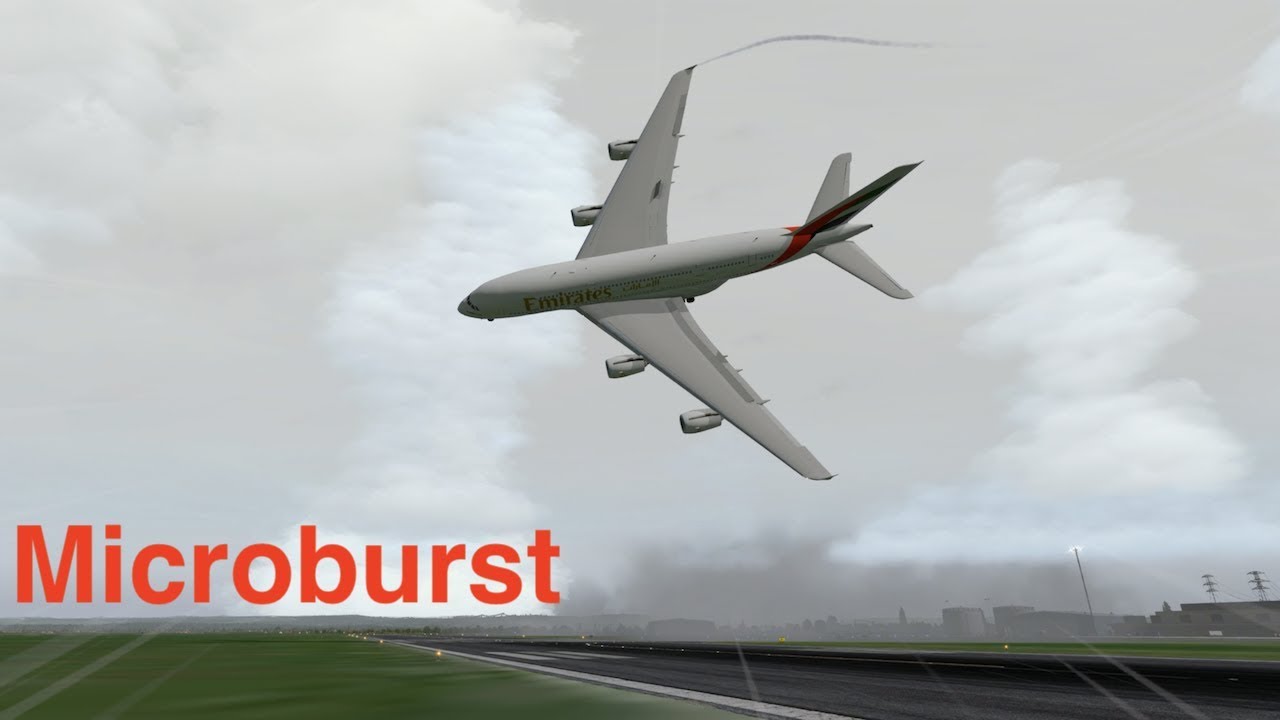The image is a computer-generated graphic depicting a dramatic and frightening aviation scenario featuring an Emirates Airbus A380 passenger jet. The aircraft is positioned perpendicular to the landing strip, with its orientation from 3 o'clock to 9 o'clock on a clock face, while the runway extends from 5 o'clock to 10 o'clock. The plane is tilted at a precarious 45-degree angle, suggesting a near-crash situation just above the airfield. The scene is set against a sky populated with various cloud formations indicating different atmospheric conditions, simulating the occurrence of a weather phenomenon. This is emphasized by the large orange text, "microburst," in the lower left-hand corner, explaining the cause of the imminent crash. The plane, which is emblazoned with Emirates livery including a red stripe and the logo, is surrounded by a hazy, grayish atmosphere. The airfield itself shows a black runway bordered by neatly cut light green grass and distant power lines. The overall depiction conveys a sense of urgency and peril.